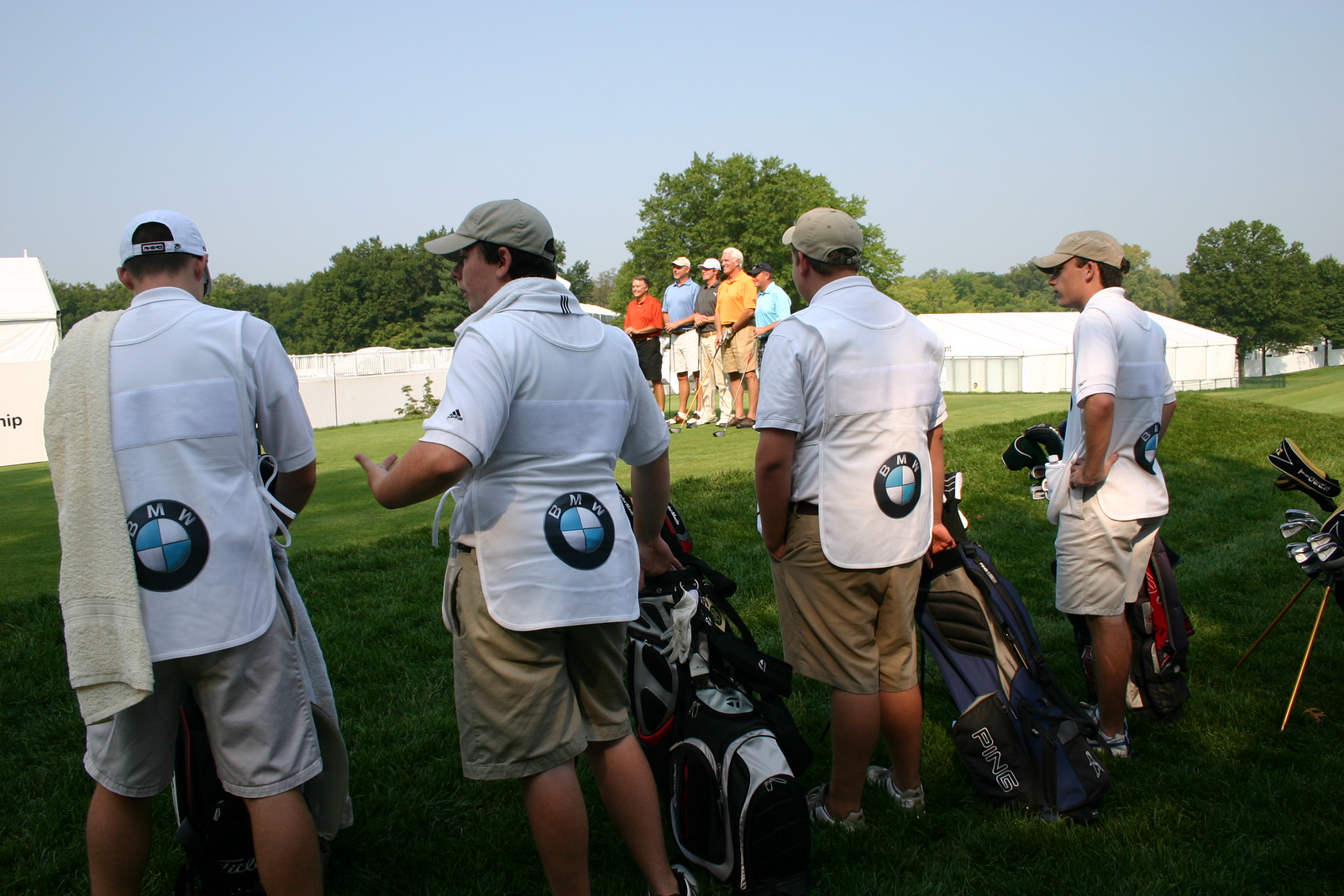This photograph captures a vibrant moment on a sunny day at a golf course, likely during a BMW-sponsored event, possibly a tournament or charity game. In the foreground, four caddies stand on lush, high grass, each with a golf bag full of clubs. They uniformly wear khaki shorts, white collared shirts, over bibs featuring the BMW logo, and baseball caps, with one caddy notably draping a beige towel over his left shoulder. Behind them, five golfers of varying ages are lined up at the tee box, dressed in vividly colored shirts—orange, blue, gray, yellow, and light blue—with some donning baseball caps. A white fence runs parallel to the golfers, flanked by white buildings that might be large tents, while a serene sky stretches above, devoid of clouds, completing this picturesque golfing scene.